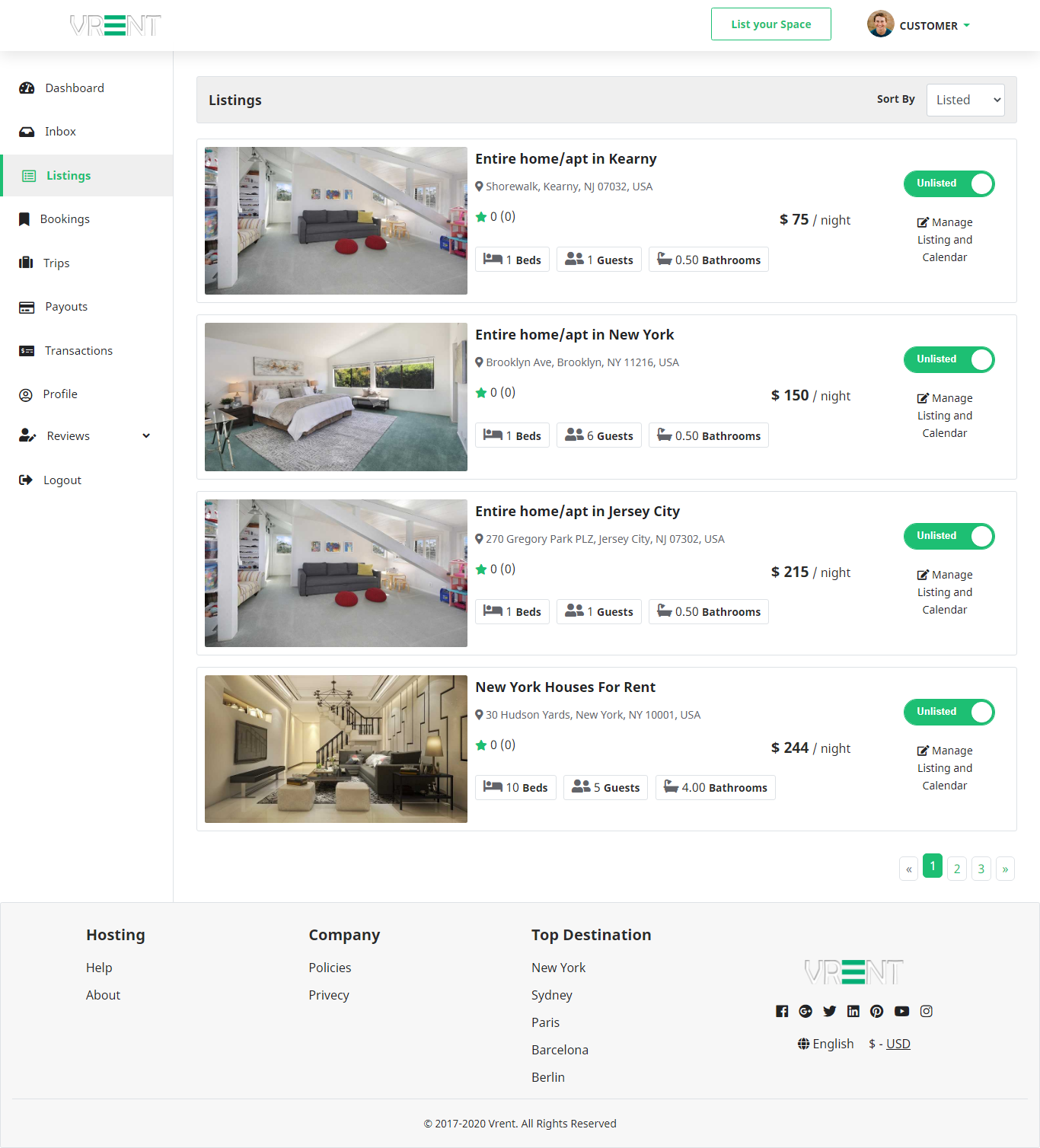This image is a cropped screenshot of the V-Rent Property Management Company webpage, depicting a section that resembles an Airbnb-style platform where listings managed by the company are displayed. At the top left corner is the V-Rent logo. Adjacent to this, on the right, is a green-outlined button labeled "List Your Space." Further to the right is a profile picture followed by the word "Customer" in bold black font, and a dropdown menu for changing the login credentials.

On the far left side of the page, there is a vertical navigation panel featuring options such as Dashboard, Inbox, Listings, Bookings, Trips, Payments, Transactions, Profile, Reviews, and Logout. Directly to the right of this panel, the main content area shows a series of property listings arranged vertically.

At the top of this section, within a gray bar, the word "Listings" is displayed on the left side. To the right of this, there is a "Sort by" label accompanied by a dropdown box currently set to "Listed." Each property listing consists of a square thumbnail image on the left, accompanied by a description of the property, its location, and the number of ratings it has received. To the right of this information, the price of the property is shown along with a toggle switch. Below each listing, there is a checkbox labeled "Manage Listing and Calendar," all of which are selected.